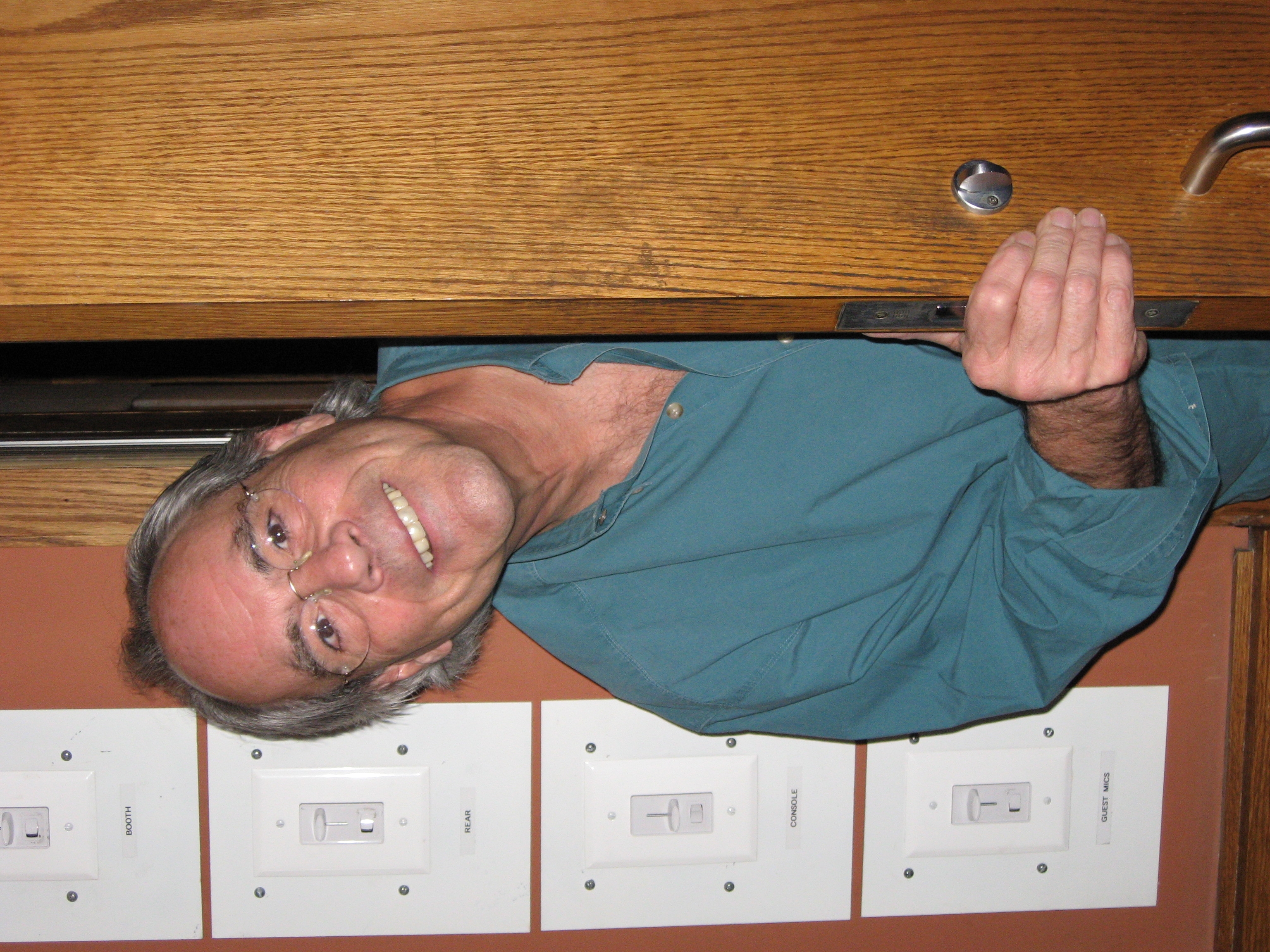The photograph captures a tan, elderly Caucasian man, likely in his late 60s or 70s, with light-colored skin and gray hair swept back from his face. He is smiling broadly, exuding excitement as he leans halfway through an open, heavy, grainy wood door that is adorned with a silver lock and handle. Gold-framed glasses with clear lenses accentuate his face, and his button-down shirt is a striking teal color with long sleeves, partially revealing a hairy arm.

The image is initially disorienting as it’s turned 90 degrees to the left, making the man appear horizontal, but his joyful demeanor remains evident. Behind him on the left side, the orange-painted wall features four white panels, each equipped with a sliding switch and a traditional flip switch below, clearly labeled "booth," "rear," "console," and "guest mics" in black writing. The setting and the man’s inquisitive yet cheerful expression suggest he is about to enter or ask permission to enter the room.